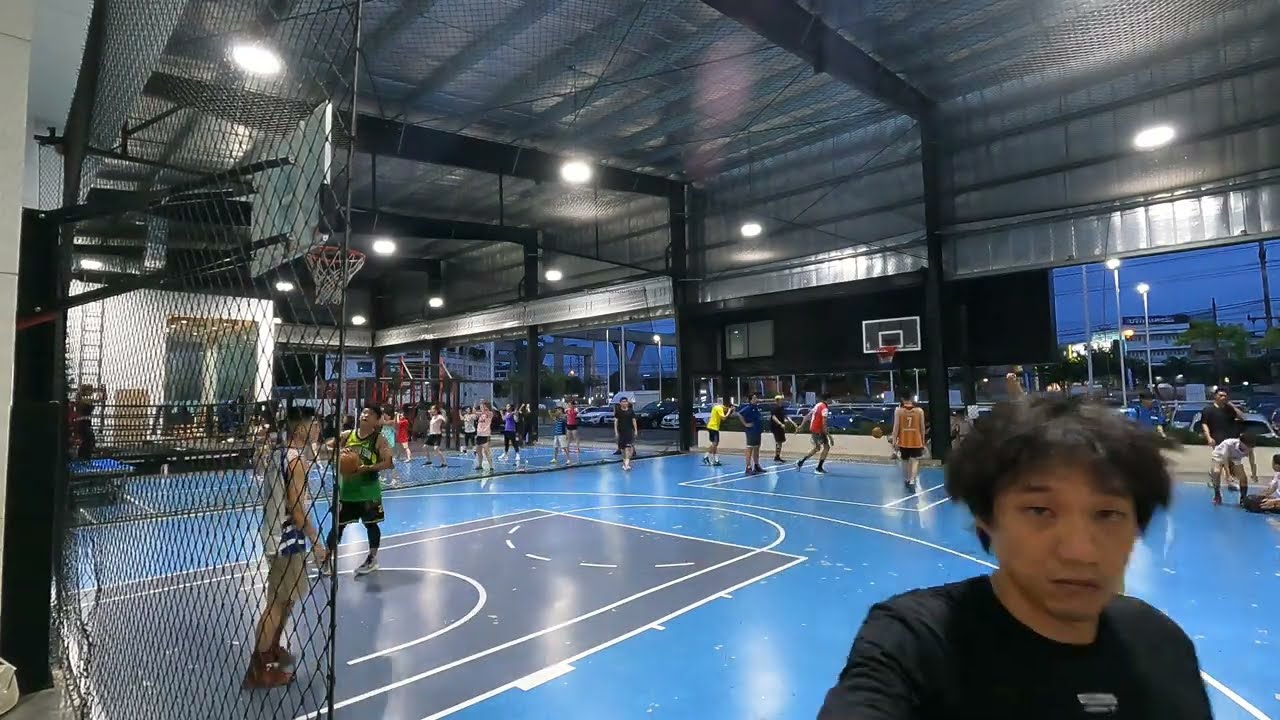In the interior of a spacious gymnasium, multiple activities are underway. The gym's floor is a mix of light blue with darker shaded inner court areas and white markings. In the center of the gym, several individuals, mostly in various colored jerseys such as green, blue, white, yellow, orange, and red, are actively engaged in playing basketball. A mesh screen has been lowered to partition a distant section of the gym, where people are performing aerobics. The ceiling is made of silver metal sheeting supported by black pillars. In the foreground, a young man with black hair, dressed in a black t-shirt, is looking directly at the camera. He adds a personal touch to the scene. To the left, two men, one in a green jersey and black shorts, and the other in a blue and white jersey with beige shorts, are involved in the basketball game. Spectators are seated on the floor near the nearest basketball court. The gym also features large openings to the outside, where the evening sky is a deep blue, hinting at the onset of night. Architectural elements visible through these openings suggest a setting possibly in Japan, enhancing the scene with a cultural context.